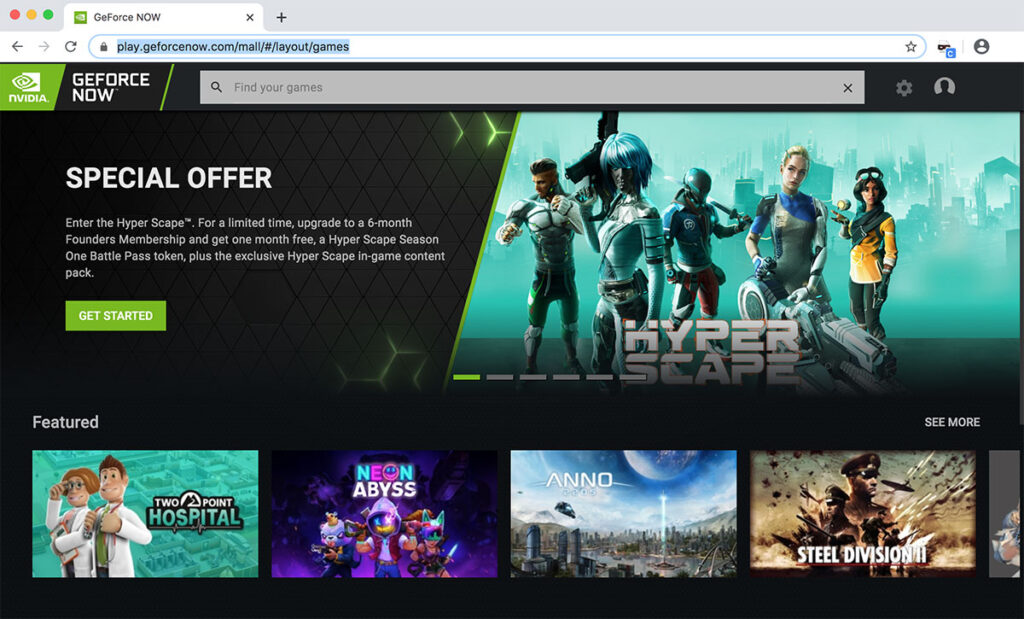The image depicts a Mac web browser window displaying the NVIDIA GeForce NOW website. In the top left corner of the browser, close icons are represented by red, gold, and green circles. The currently open tab is GeForce NOW by NVIDIA. Below the address bar, the interface features a black background, with the green and white NVIDIA logo and "GeForce NOW" text situated at the upper left corner. A large, centralized search bar is prominently displayed at the top center, flanked to its right by the settings icon and user profile icon.

The screen's central area is split. On the left, there's a "Special Offer" section with a "Get Started" button. To the right of this, an eye-catching cover art for the game "Hyper Scape" (or "Hyperscape") is shown, depicting five characters. 

At the bottom of the page, a "Featured Games" section is visible. On the bottom left is an icon for "Two Point Hospital," followed by "Neon Abyss," "Anno," and "Steel Division 2" as you move to the right. Above the "Steel Division 2" icon, there is a clickable "See More" button to explore additional games.